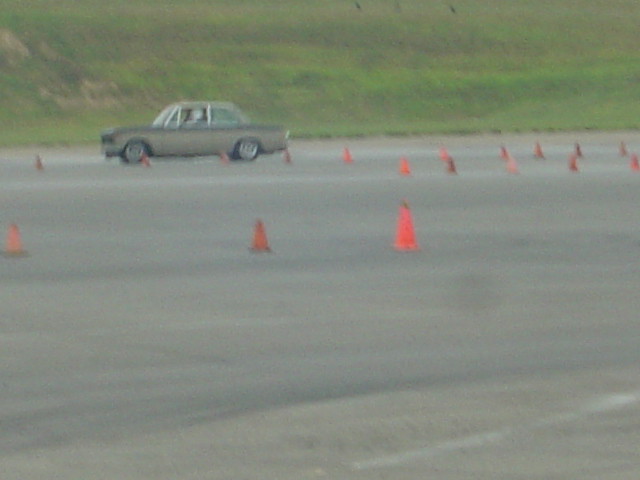This slightly blurry color photograph, possibly taken years ago, depicts an outdoor driving obstacle course. The course is set up with an array of bright orange, highlighter-colored cones arranged in a series of patterns. The grayish-tan car navigating the course appears to be from the mid to late 1960s, indicated by its shape and style. The vehicle features matching colored hood and sides, black tires, and shiny silver hubcaps. A driver, who is wearing a white helmet, is visible inside the car. The setting includes a road with a few white lines and an old, empty parking lot. In the background, there's a grassy hill that occupies the upper portion of the scene.